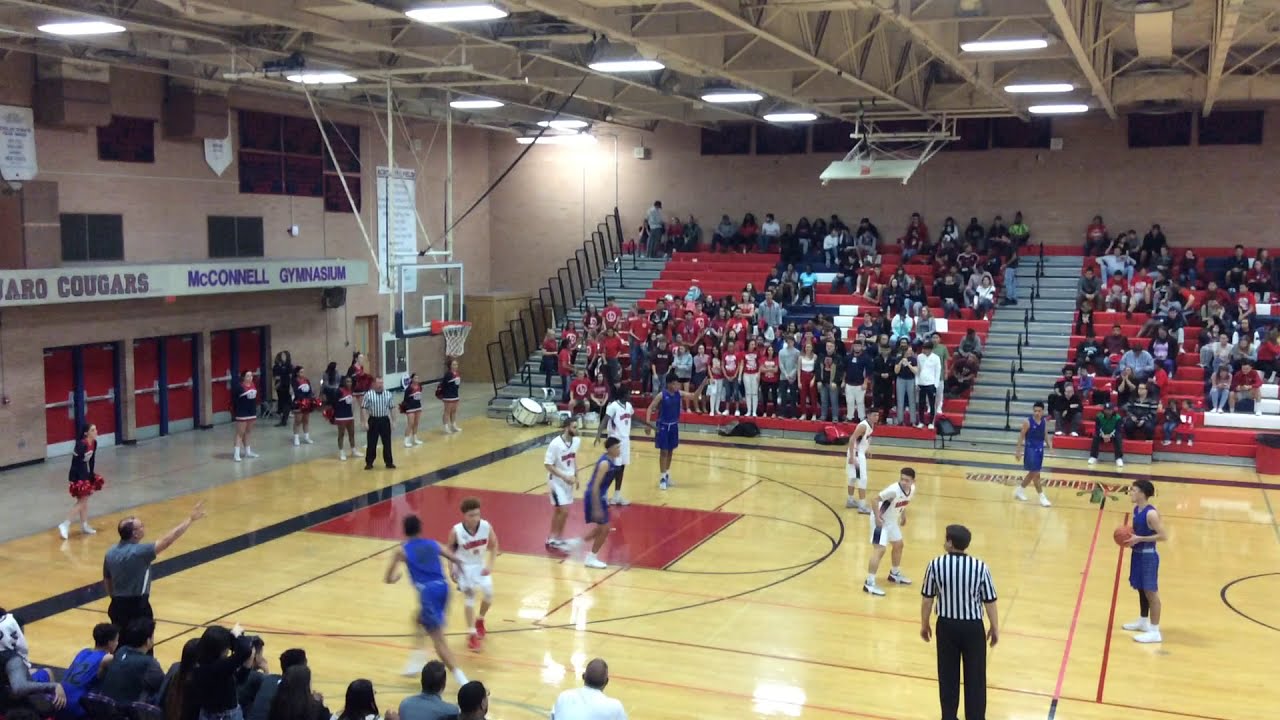The photograph captures an intense high school basketball game inside the McConnell Gymnasium, showcasing the dynamic energy of the gym. The game features two teams: one dressed in blue shorts and blue sleeveless jerseys, and another in white shorts and white jerseys, all sporting white sneakers. The light wooden gym floor is marked with red stripes and black circles. Above the court hangs two white and orange basketball hoops. The gymnasium seats are painted silver and red, with the crowded bleachers filled with animated spectators. Cheering loudly, fans can also be seen on the opposite side of the gym, which is constructed of brown brick and features three red double doors. High up in the stands, where the photo appears to be taken from, you can glimpse the cheerleaders on the left side wearing red and black uniforms. A prominent white banner hangs above the court, adorned with the words "Cougars McConnell Gymnasium," set against a background of fluorescent lighting and rafters. The vibrant atmosphere and detailed elements come together to vividly depict the excitement of the high school basketball game in progress.